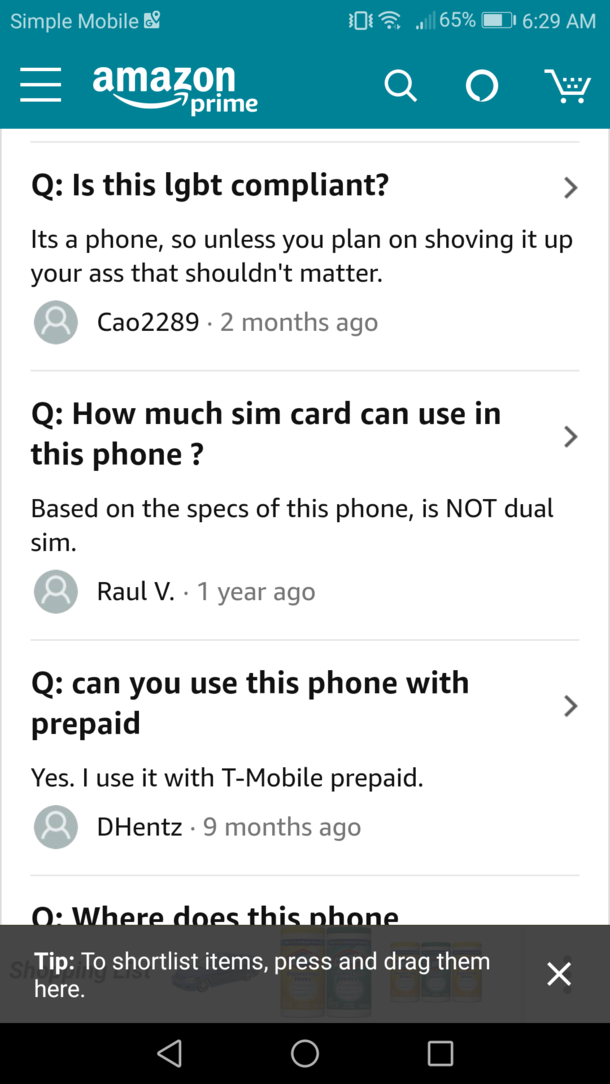In this screenshot, we see a bluish-green banner occupying the top section. In the upper left corner, small light green text reads "Light Teal, Symbol Mobile." To the right on the upper screen, there is a Wi-Fi icon showing two out of five bars, a battery icon indicating 65% charge, and the time displayed as 6:29 AM in the upper right corner. Beneath these icons on the same banner, the Amazon Prime logo appears in white, flanked by a white magnifying glass, a white circle, and a white shopping cart icon.

Below the banner, bold black text poses the question, "Hue, is this LGBT compliant?" The highlighted reply underneath, from user cao2289, states, "It's a phone, so unless you plan on shoving it up your ass, that shouldn't matter." This reply was posted two months ago. The content is casual and a bit flippant in tone.